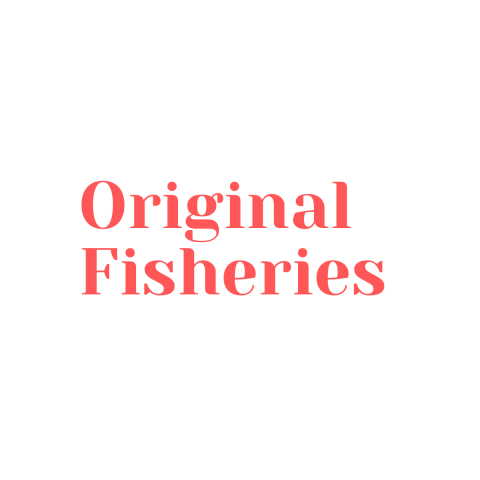The image features a minimalistic design, likely an advertisement for a company named "Original Fisheries," displayed against a solid white background. The text is arranged in two lines, with "original" on the top line and "fisheries" on the bottom, both left-justified. The letters are a light reddish color, with the initial "O" in "original" and "F" in "fisheries" capitalized while the rest of the letters are lowercase. The faded and subdued appearance of the text suggests a vintage or retro quality, possibly reminiscent of an older company or something sourced from an old newspaper or magazine. There are no other elements—no logos, images, additional text, or punctuation—making the simplicity of the design noteworthy.